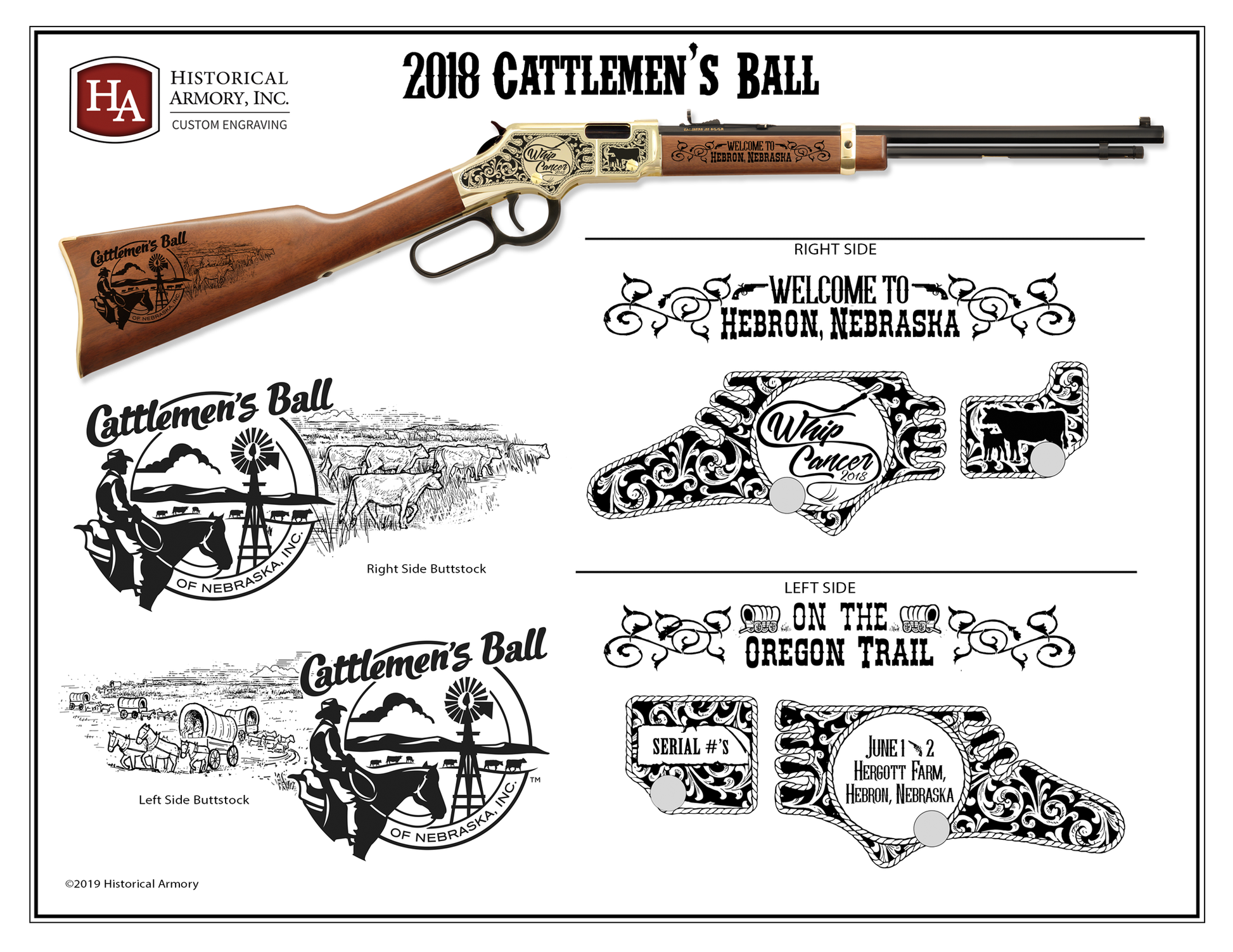This image features a detailed diagram of a rifle prominently displayed in the center. The rifle itself is an intricate blend of dark wood, gold accents, and a black barrel, presenting a striking appearance. Above the rifle, the caption "2018 Cattleman's Ball" is prominently displayed, indicating its association with the event. In the top left-hand corner, the logo for "Historical Armory Ink" set against a red background, stands out, accompanied by the text "custom engraving" beneath an underline.

On the stock of the rifle, an engravement shows a man seated, looking at a windmill, and the text "Welcome to Hebron, Nebraska" is etched towards the front of the gun. The right side of the rifle's buttstock features the engravings "whip cancer 2018" and "whip conserve 2018." On the left side, the "Cattleman's Ball" symbol reappears on the buttstock along with "left side on the Oregon Trail." Towards the bottom of the image, "June 1-2, Haggard Farm, Hebron, Nebraska" is inscribed, denoting the specifics of the event.

Beneath the rifle, various images are depicted to represent the detailed engravings and symbols present on the actual gun. This advertising poster effectively showcases the exquisite design options available for rifle customization, curated by Historical Armory Ink.